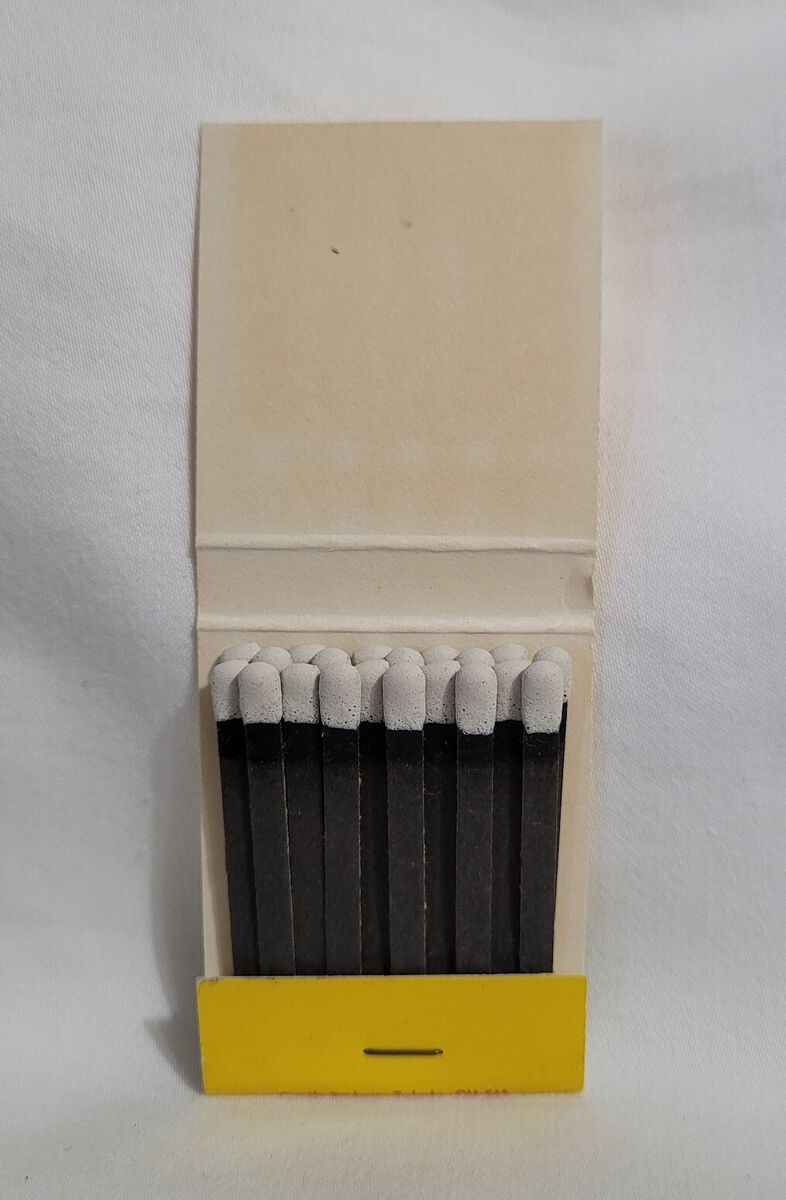This image captures an open yellow matchbook set against a white background. The matchbook contains 20 matches, each with black stems and white heads, all intact and unused. The yellow cover is folded over the bottom of the matchsticks and secured by a staple. The inside cover, originally white, appears aged and stained, showing visible imprints and light spots where the match heads have rested over time. The overall appearance suggests the matchbook is old, evidenced by the tan, stained interior that contrasts with the bright yellow exterior.